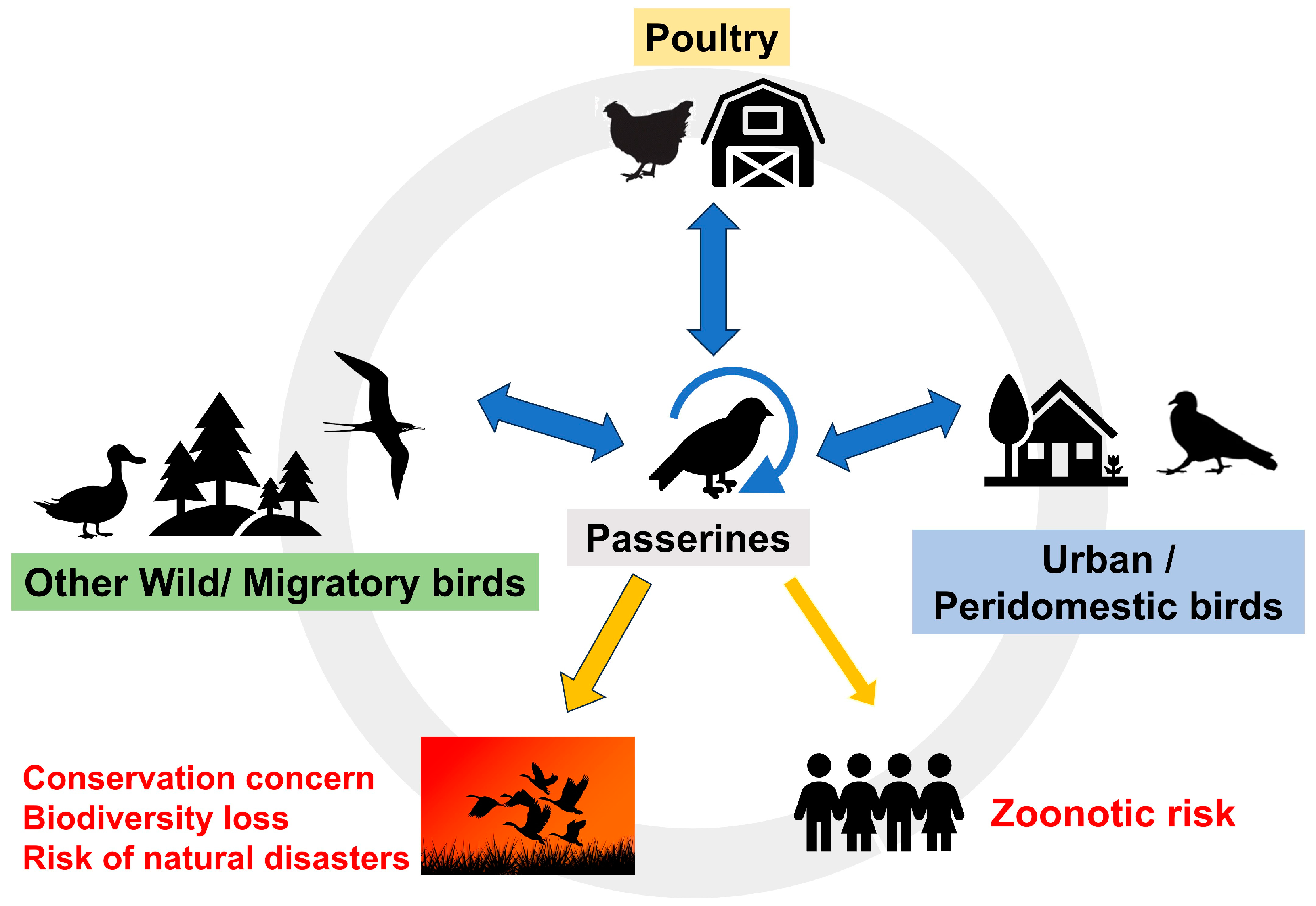The image is a detailed chart likely from a presentation slide or textbook, depicting various challenges faced by bird species. Set against a white background with a central gray circle, the focal point is a black silhouette of a bird labeled "passerines" in a gray banner. Numerous blue arrows radiate from this central bird to different sections around the circle, resembling a clock face.

At the 12 o'clock position, the chart highlights "poultry" with an illustration of a chicken and a barn. Moving clockwise to 3 o'clock, the chart includes "urban peri-domestic birds," depicted by a bird beside a house. Next, at 5 o'clock, the focus shifts to "zoonotic risk," illustrated with icons of four people in red text. Continuing to 7 o'clock, the section addresses "conservation concern, biodiversity loss, risk of natural disasters," marked by silhouettes of geese against an orange background. Finally, at 9 o'clock, labeled "other wild migratory birds," the chart shows silhouettes of a duck, evergreen trees, and a bird with a large wingspan, possibly an osprey, against a green box.

The arrows from the central passerine bird to these sections underline the interconnected nature of these issues, emphasizing zoonotic risk, biodiversity loss, and the ecological challenges tied to various bird species.